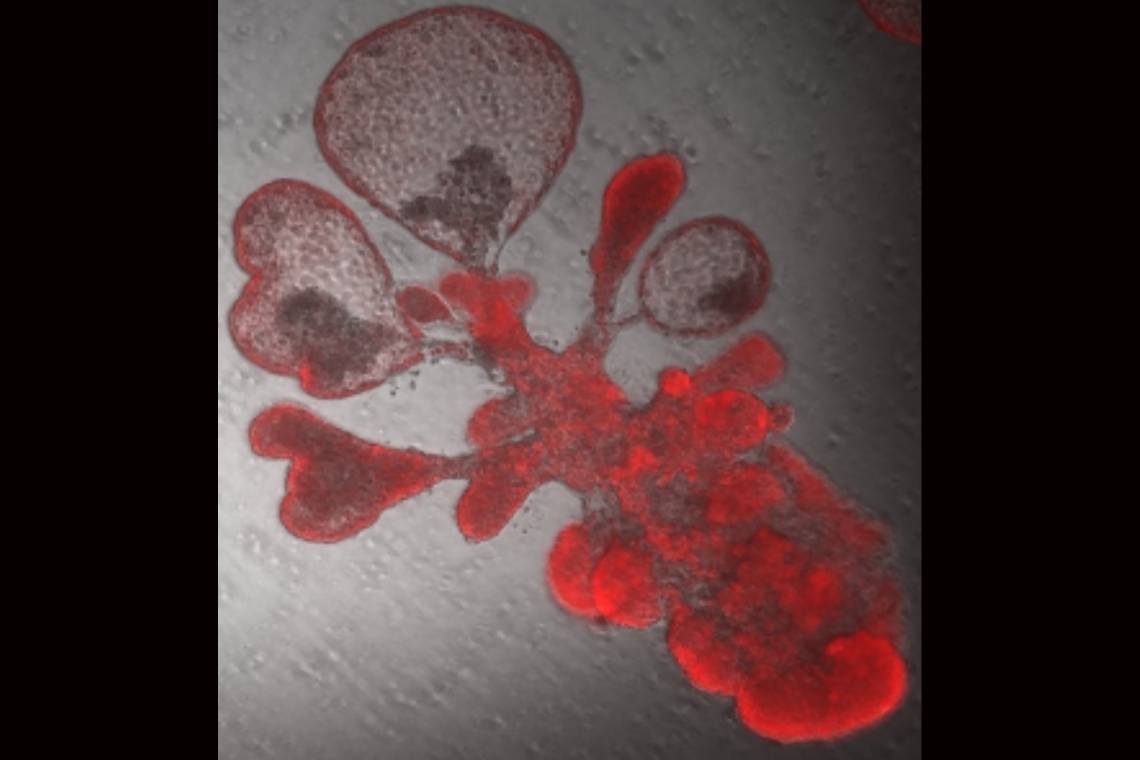The image appears to resemble a highly magnified view, akin to a microscope slide, showcasing an organic formation that suggests bacterial growth or cellular structures. Dominating the image is a substantial red splotch with overlapping, irregularly shaped fields, branching out in a way that evokes flowering or spreading bacterial colonies. These forms are primarily round and irregular, with tiny dots populating their interior, adding a textured appearance.

Positioned above the main splotch are three translucent shapes—a circle, a teardrop, and a heart—all edged in red but featuring mottled gray-and-white interiors. The larger lobed splotch on the left extends into a smaller, finger-like projection. The background is a gray, metallic surface adorned with bubbled or rippled textures, reminiscent of dew or water droplets, though more likely representing a textured, gray ambiance. This combination of detailed, organic shapes and textural elements creates a visually intricate and complex scene.